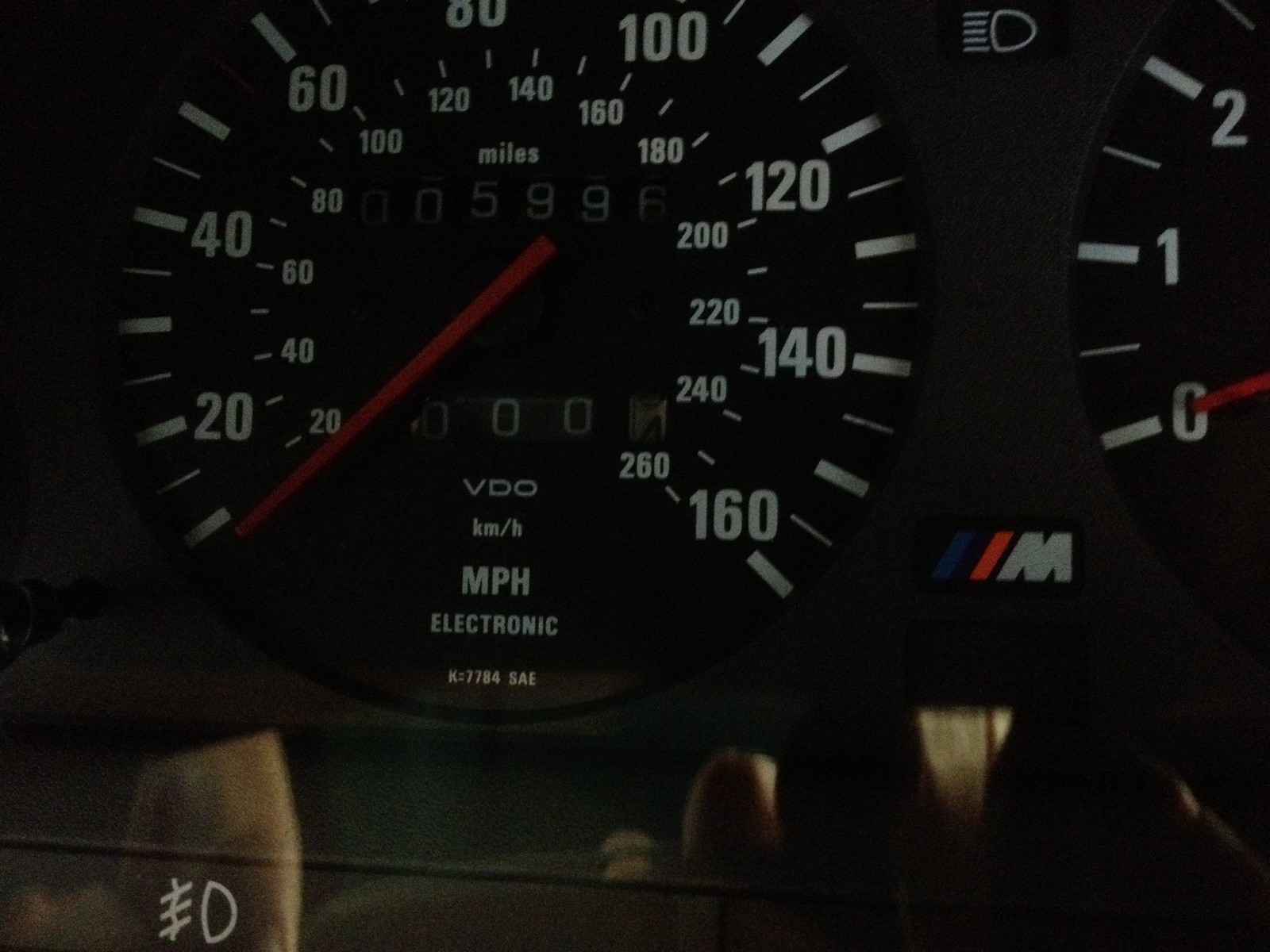This is a close-up photo of a BMW M line speedometer, highlighting a blend of precision and design. The image shows a classic analog dial with a red needle resting at zero, indicating the car is off. The speedometer features white numbers displaying speeds from 0 to 160 miles per hour in increments of 20. The inner ring also shows speeds in kilometers per hour, ranging from 20 to 260. The vehicle's mileage is currently at 5,996, with VDO, kilometers per hour, MPH, and electronic labels visible under the numerical displays. To the right of the speedometer is the distinctive BMW M emblem with blue and red hashtags surrounding a white 'M', marking it as part of the M-Class series. In the upper right corner, there's a partial view of the tachometer, also at zero, showing the numbers 0, 1, and 2. The image captures some reflections off the plastic casing that houses these instruments, adding a layer of depth to the photo. Additionally, white icons for the headlights and fog lights are visible, although unlit.